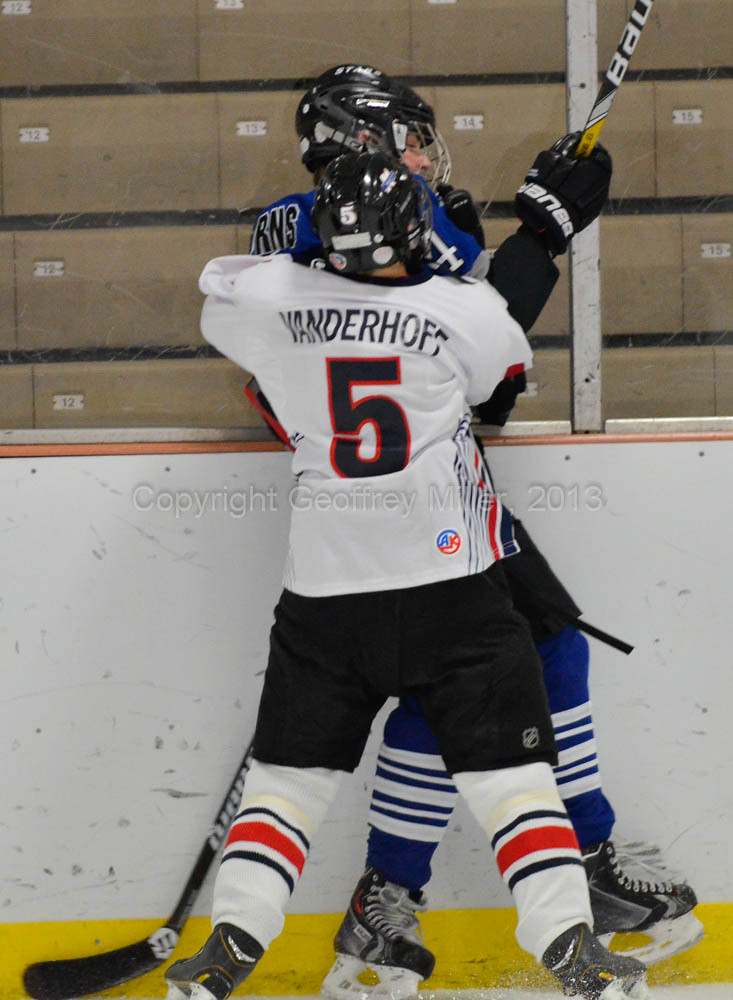Inside a hockey rink, two hockey players are engaged in an intense struggle against the protective glass wall. The bottom half of the wall is white with a yellow strip, while the top half is transparent glass. In the background, a series of boxes are labeled sequentially from left to right: 12, 13, 14, and 15.

The player being pushed against the glass appears slightly taller and is wearing a dark blue jersey and pants, black shorts, a black helmet, and blue shin guards with white stripes. His right arm is raised, holding his hockey stick pointed to the top right.

The player exerting the pressure wears a white jersey with the number 5 prominently displayed on the back, outlined in red. His uniform includes black shorts, white pants with red stripes, white shin guards, and a black helmet. The name "Van Der Hoof" is partially visible above the number 5, though it is difficult to read fully due to the crumpled fabric.